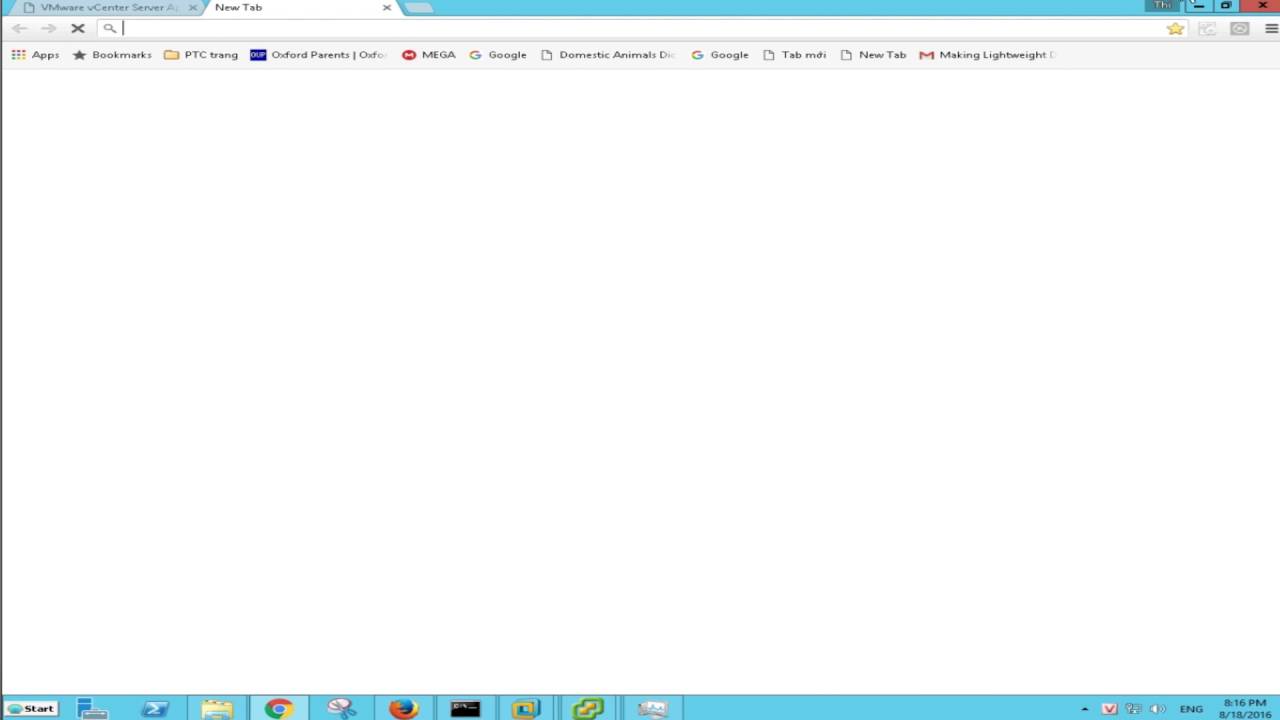### Detailed Caption for the Image

The screenshot features a web browser window with multiple elements visible. 

- **Tabs**: 
  - At the top-left corner, two tabs are present. The inactive tab is labeled "VMware vCenter server," followed by an unreadable text starting with 'A.' 
  - The active tab is simply labeled "New Tab."

- **Window Controls**:
  - To the far right are the standard window controls:
    - Minimize
    - Maximize
    - Close (a red button with an 'X' in it)

- **Search Bar**:
  - Positioned just below the tabs, the search bar is empty except for a blinking cursor.
  - On the left of the search bar is a magnifying glass icon.
  - On the right of the search bar are several icons:
    - A gold star, likely for 'Favorites.'
    - A stopwatch-like icon.
    - A circle with a dot in the middle.
    - A hamburger menu (three horizontal lines).

- **Favorites Bar**:
  - Below the search bar, a row of favorite links/icons is visible:
    - "Apps"
    - "Bookmarks" with a star icon.
    - A folder labeled "PTC TRANG."
    - A blue icon labeled "Oxford Parents."
    - A red circular icon labeled "Mega."
    - A Google logo labeled "Google."
    - A plain page icon labeled "Domestic Animals," with a trailing unreadable word starting with 'D.'
    - Another Google logo labeled "Google."
    - A plain page icon labeled "Tab," with an unreadable trailing word starting with 'M.'
    - A blank page icon labeled "New Tab."
    - A Gmail icon labeled "Making Lightweight."

- **Main Area**:
  - The bulk of the screenshot is taken up by empty white space below the favorites bar.

- **Taskbar (Bottom Edge)**:
  - From left to right, several icons are present:
    - A gray button with a blue icon labeled "Start."
    - An unrecognized gray-blue icon.
    - A Manila folder icon.
    - Google Chrome icon.
    - Snip tool (scissors inside a circle).
    - Firefox icon.
    - A black rectangular icon.
    - An icon of a yellow square atop a blue square.
    - An icon of a green irregular shape with two yellow rectangles inside.
    - An icon of a computer monitor with a PC beside it.
    - A shield icon marked with a 'V.'
    - An indistinguishable icon.
    - A speaker icon for sound.
    - An indicator showing "E G" presumably for English language settings.
    - The time displayed as "8:16 PM."
    - The date displayed as "18.2016."

This comprehensive caption provides a detailed description of all visible elements within the screenshot.